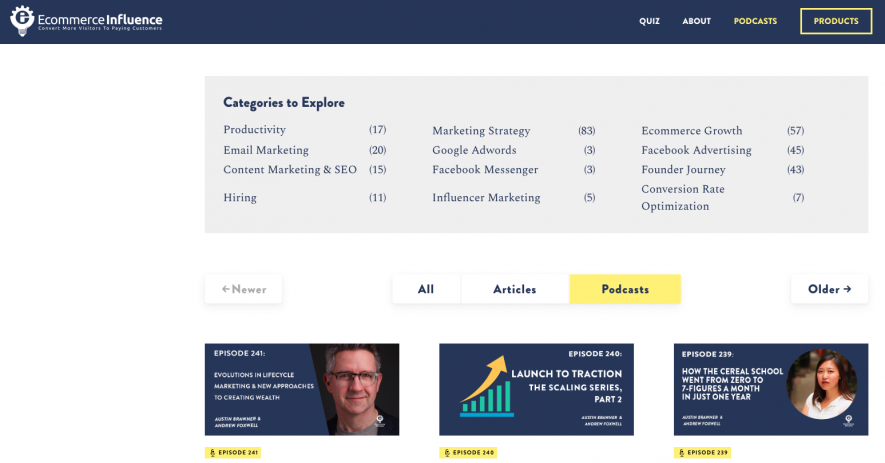The image depicts the homepage of the E-commerce Influence website. In the upper left corner, there is an icon resembling a light bulb with a lowercase "e" inside it. Adjacent to this icon, the text "E-commerce Influence" is prominently displayed, with "Influence" in bold white letters. Underneath this, there's some smaller, indistinct writing.

On the right side of the blue banner that spans the top of the page, there is a gold-highlighted text that reads "Quiz about Podcast." Adjacent to this, another label saying "Products" is enclosed within a gold-trimmed rectangle. 

Below the blue banner, there is a section of white space followed by a long gray rectangular box that contains the heading "Categories to Explore" in bold text. Within this gray box, there is a list of categories including:
- Productivity
- Email Marketing
- Content Marketing
- SEO
- Hiring
- Marketing Strategy
- Google AdWords
- Facebook Messenger
- Influencer Marketing
- E-commerce Growth
- Facebook Advertising
- Calendar Journey
- Conversion Rate Optimization

Each category is accompanied by a number in parentheses.

Below this section, on the left side, the word "Newer" along with a left-facing arrow is displayed. In the central part of this section, "All Articles and Podcasts" is highlighted in yellow. On the right side, the word "Older" is shown.

At the bottom of the page, there are media images featuring people's faces. The first and last images have people's faces, while the middle image appears to display a graph with an arrow pointing upwards.